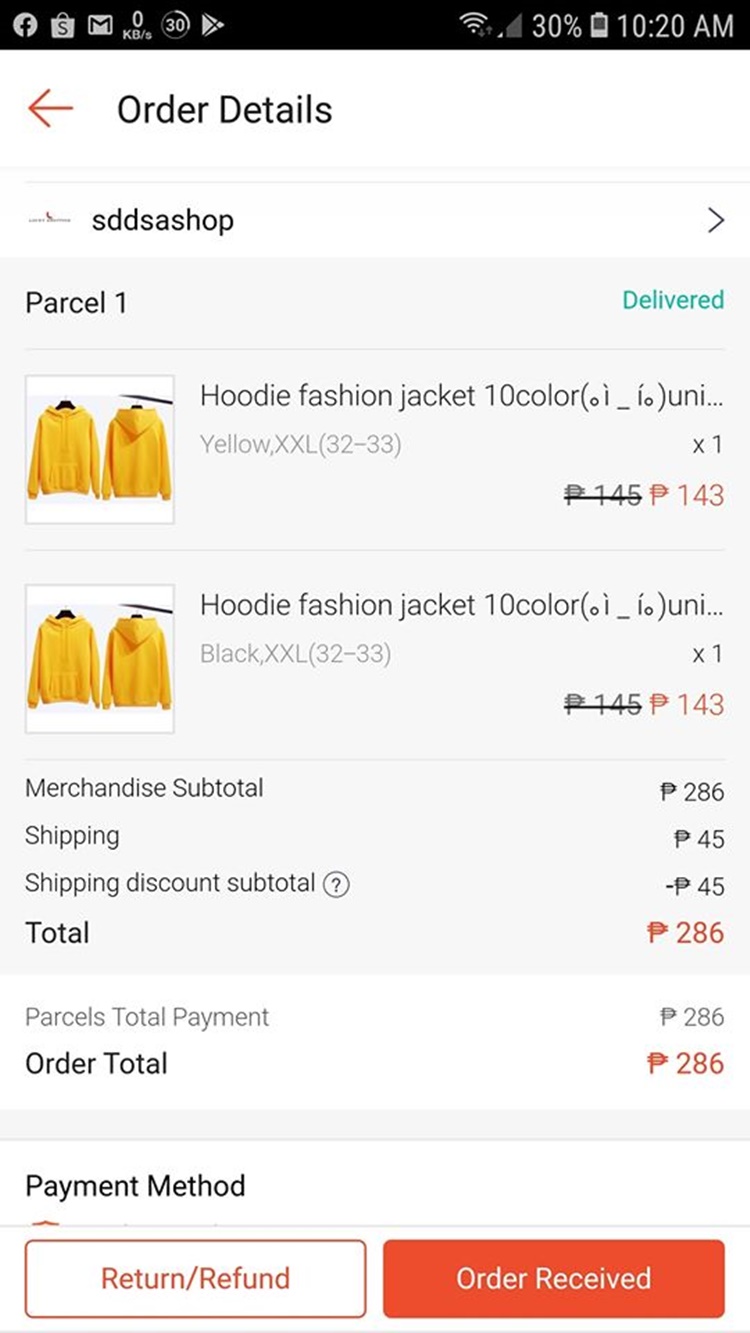An image showcases a smartphone screen against a white background. The screen displays details of an order from "SDDSA shop" with the label "Parcel One." The status of the order is shown as "Delivered," highlighted in green.

**Product Details:**
1. **First Product:** A hoodie fashion jacket, available in ten colors. The selected version is in yellow, size XS (32-33). The price is P143, originally P145, with the previous price struck through. 
   - Accompanying the description are images of two yellow jackets on the left side of the screen.
   
2. **Second Product:** The same hoodie fashion jacket in black, also in size XS (32-33) and priced at P143.
   
**Order Summary:**
- **Merchandise Subtotal:** P286
- **Shipping:** P45
- **Shipping Discount:** -P45
- **Total:** P286
- **Parcel Total Payment:** P286
- **Order Total:** P286

At the bottom of the screen, there are two buttons. The one on the bottom left, labeled in orange, reads "Return or Refund." The button on the bottom right, also in orange, reads "Order Received."